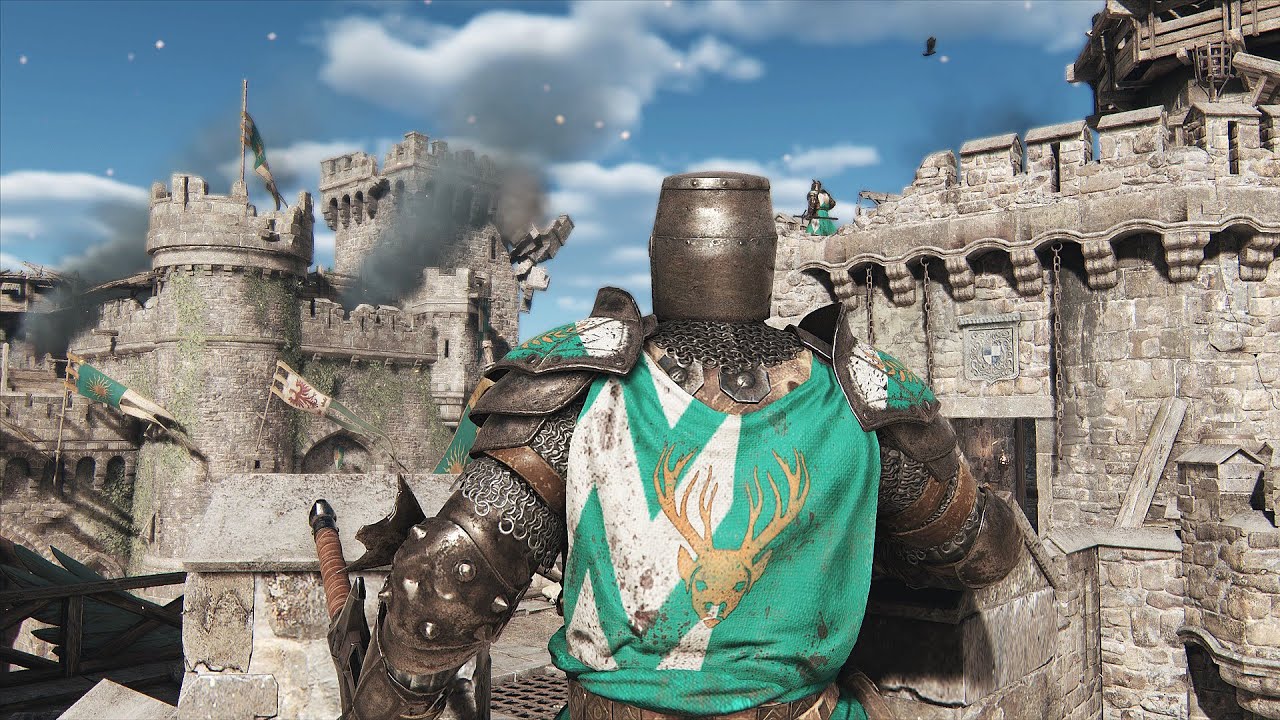In this detailed image, a medieval knight is standing in the foreground, facing a besieged castle. The sky is cloudy yet bright, indicating daytime. The castle, displaying various medieval architectural features, occupies the background. The knight wears metallic armor and chainmail, draped over with a white and green cloth adorned with a gold emblem of a reindeer buck with antlers. He also has spiky elbow pads and holds a sword by the sheath, with the handle pointing outward towards a battlefield. The cloth is notably split in half with a green lightning pattern on the left side.

Atop the right section of the castle stands another knight, mirroring the stance and attire of the foreground knight, also holding his sword by the sheath. Below this knight, the castle walls appear damaged and crumbling, with grey smoke rising, characteristic of an ongoing siege. Various flags are visible, including one depicting a red bird and another with a sun on a green background.

In the top right corner of the image, a bird is flying, adding to the dynamic scene. A shadow is cast at the bottom left, indicating the two sections of the castle visible are part of a larger fortification system. Despite the battle scene, the sky remains semi-clear, enhancing the contrast between the serene environment and the turmoil below.